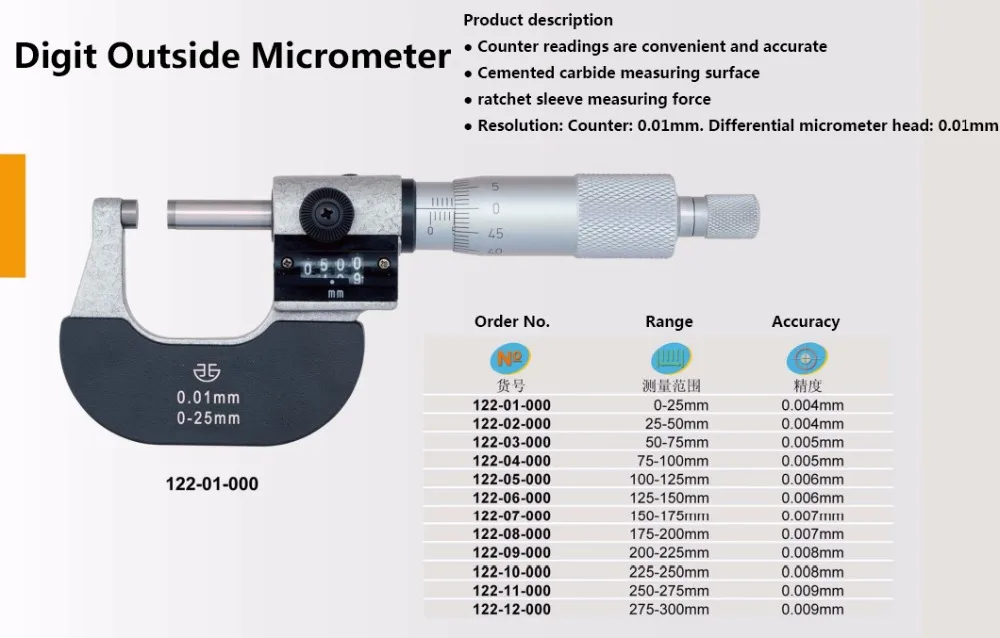The image depicts a detailed diagram of a digit outside micrometer, likely intended as a demonstration or product overview. At the top left corner, it features a bold heading "Digit Outside Micrometer." Surrounding the image, various product descriptions are provided in bullet points, highlighting its key features: convenient and accurate counter readings, a cemented carbide measuring surface, ratchet sleeve for measuring force, and a resolution counter of 0.01 mm with a differential micrometer head of 0.01 mm.

The instrument itself has a U-shaped body that resembles a gun, crafted from steel or iron, with multiple screws and numeric scales etched on its surface. A digital display on the device shows measurements in millimeters (mm). The handle is fitted with an adjustable dial, inscribed with measurements ranging from 0.01 mm to 0.225 mm. 

Beneath the image, there are columns of text detailing order number, range, and accuracy specifications, some of which include annotations in an Asian script. The order numbers span from 122-01-000 to 122-12-000, covering a measurement range from 0-25 mm to 275-300 mm, with corresponding accuracy varying from 0.004 mm to 0.009 mm. The comprehensive layout and detailed specifications indicate this diagram is a meticulously crafted guide to the micrometer’s functionality and ordering information.